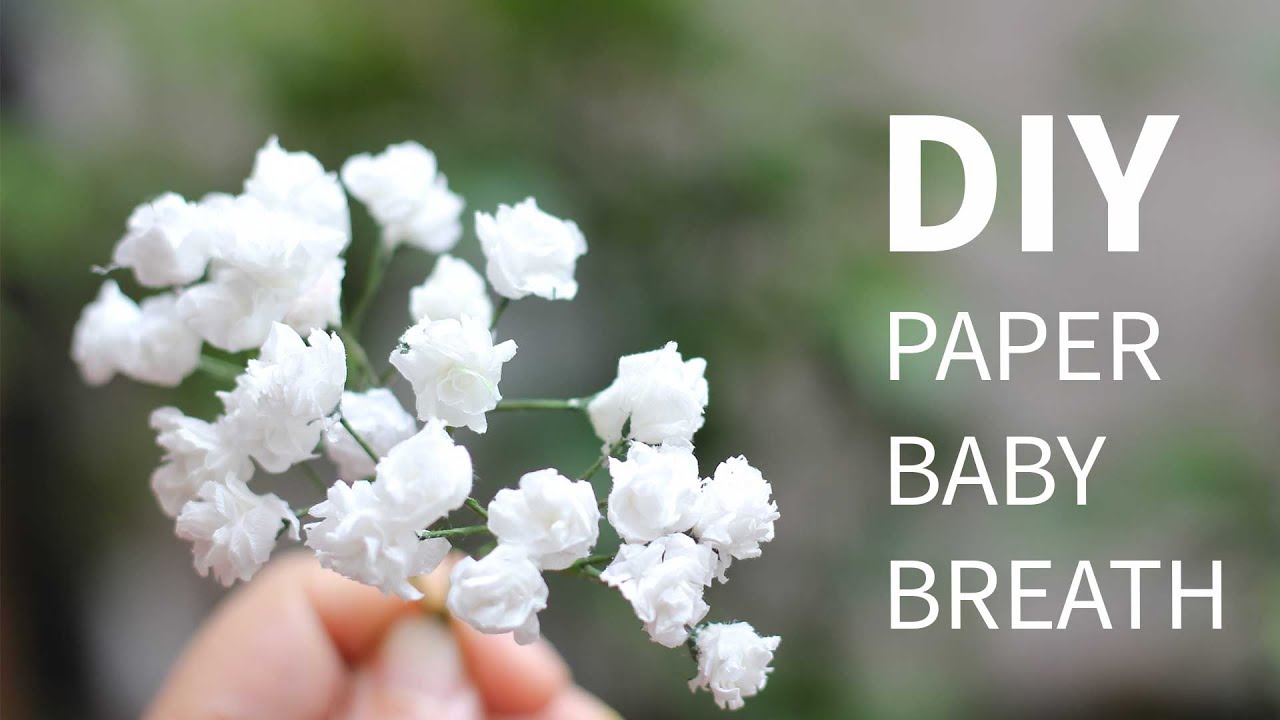This is a detailed and descriptive photographic-style drawing of a sprig of baby’s breath flowers, captured outdoors during the daytime. The background is intentionally blurred, hinting at green vegetation and possibly gray walls or ivy leaves, providing a natural yet indistinct backdrop. The main focus of the image is on the sprig of baby’s breath, which features around 16 small and delicate white blossoms adorning green stems.

The sprig is being held by the fingertips of an individual with a slightly out-of-focus Caucasian hand, positioned on the left side of the image. Most of the blossoms are in sharp focus, though some on the left edge trail into a slight blur. The image transitions from a dark black in the bottom left corner to a mix of white and light green in the top right, creating a gradient effect.

Superimposed on the right side of the image, in large, bold white letters, are the words "DIY PAPER BABY BREATH," with "DIY" being the most prominent, followed by "PAPER," "BABY," and "BREATH" in slightly smaller font. The text suggests this could be an introductory page for a craft book or a YouTube tutorial.